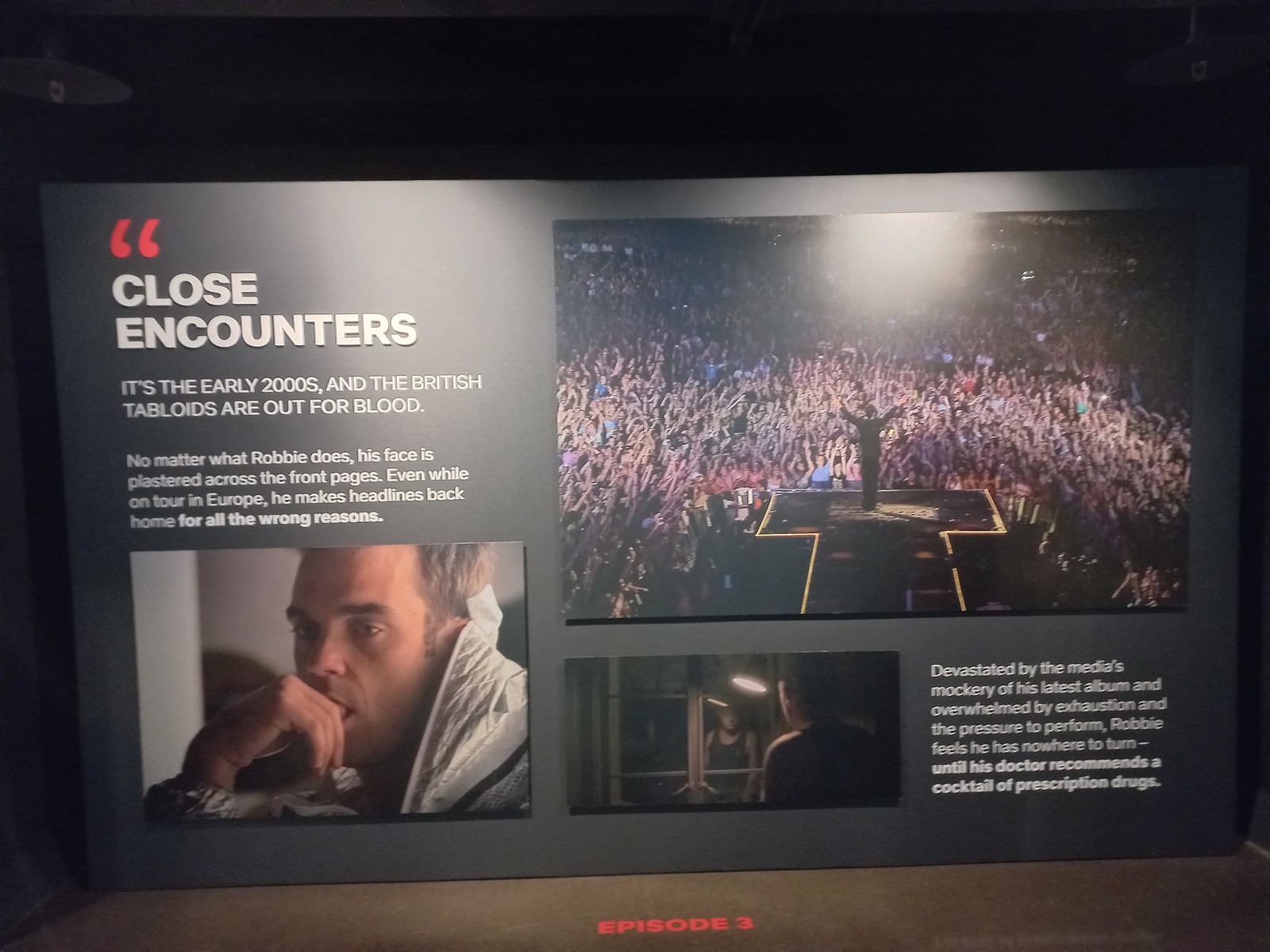The photograph captures an indoor poster titled "Close Encounters" in bold, white letters positioned at the top left corner. Below that, accompanying text in smaller white capital letters reads, "It's the early 2000s and the British tabloids are out for blood." The narrative continues in standard capitalization, stating, "No matter what Robbie does, his face is plastered across the front pages. While on tour in Europe, he makes headlines back home for all the wrong reasons," with "for all the wrong reasons" emphasized in bold. 

In the lower left-hand corner, there is a close-up image of a serious-looking white man with his hand to his mouth, wearing a white jacket. Adjacent to this, another image depicts a man standing on stage, gazing out at a sea of people with their hands raised. Amidst this visual storytelling, an inset photo shows a man looking into a mirror, accompanied by the text: "Devastated by the media's mockery of his latest album and overwhelmed by exhaustion and the pressure to perform, Robbie feels he has nowhere to turn until his doctor recommends a cocktail of prescription drugs." At the bottom of the poster, the text "Episode 3" is prominently displayed in orange, signifying its sequence in a series.